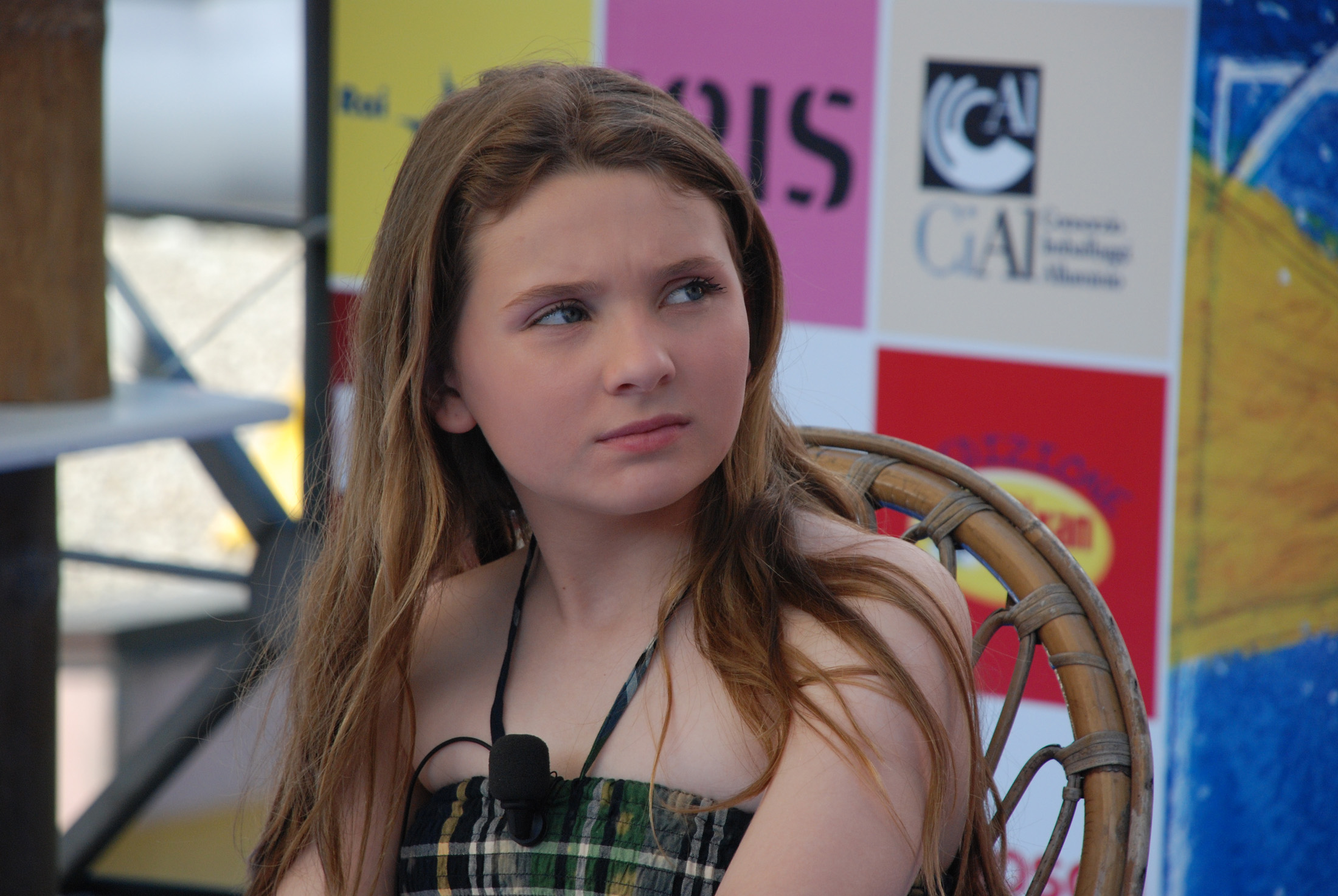In this detailed image, we see a young girl with long, orange-brown hair cascading down to her chest. Her gaze is directed up and to the right, revealing a contemplative expression as she seems to be engaged in conversation. She is seated centrally and comfortably in a woven, wicker chair that sports shades of light and dark brown. The girl is dressed in a distinctive halter top that ties at the back of her neck, boasting a plaid pattern in greens, whites, yellows, and hints of blue. Clipped to the front of her top is a microphone, indicating that she might be part of some event or interview. The background is filled with a grid of colorful advertisements suggesting sponsorship, including squares in yellow, purple, white, and red, arranged in rows of three. Some of the text on these ads is partially legible, with one possibly spelling out "G-A-I" or "C-A-I." Additionally, a blue and yellow design can be seen on the right side of the image, adding to the vivid and eclectic atmosphere of the scene.